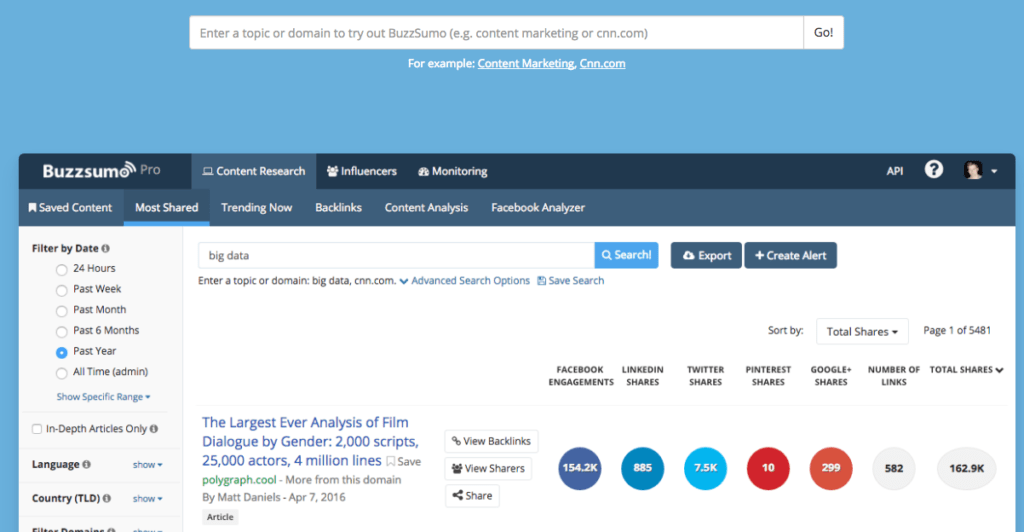### Detailed Caption for BuzzSumo Pro Interface Screenshot

The screenshot captures the interface of BuzzSumo Pro, a content research tool, showcasing various features and options for exploring and analyzing online content. The overall background is a soothing sky blue color, with a prominent white section in the center that houses the main functionalities.

At the very top of the screen, within the blue section, there's an input field prompting users to "Enter a topic or domain to try out BuzzSumo," followed by examples like "content marketing" or "cnn.com." Beside this prompt, there's a black "Go" button on the right-hand side. Directly beneath, on a nearly black banner, similar examples are repeated in white text.

The main white section at the center features the BuzzSumo logo in white, and directly to the right, the selected tab "Content Research" is marked, which includes an icon of a laptop. Adjacent to this tab, there are unselected labels "Influencers" and "Monitoring," both in white text.

Below these tabs, a lighter gray-green bar extends across, displaying menu labels such as "Saved Content," "Most Shared," "Trending Now," "Backlinks," "Content Analysis," and "Facebook Analyzer." The label "Most Shared" is currently selected, indicated by a blue underline.

The interface's left vertical column is dedicated to filtering and refining the content based on specific criteria. Options include filtering by date ranges like the past 24 hours to all time, with "the past year" currently selected in blue. Additional filters include "Language," "Country," and another obscured option, each paired with a "Show" button featuring a blue down arrow.

Central to the display is a white text area where a user has entered the term "big data." To initiate the search, there's a blue "Search" button adjacent to it. Further to the right, there's a dark gray "Export" button with a download icon, and a white "plus" sign button labeled "Create Alert."

Underneath, a repeated prompt advises to "Enter a topic or domain Big data," giving the CNN example once again. Below this, in dark blue hyperlinked text, is an example research result titled "The largest ever analysis of film dialogue by gender: 2,000 scripts, 25,000 actors, 4 million lines," credited to "Polygraph.cool" in green text. To the right of this example, actionable buttons include "View backlinks," "View sharers," and "Share."

Aligning horizontally across the page are black labels for engagement metrics: "Facebook engagement," "LinkedIn shares," "Twitter shares," "Pinterest shares," "Google shares," "Number of links," and "Total shares." Overseeing these metrics, there's a sorting option with a white button labeled "Total shares" in black text and an indicator showing "Page 1 of 5481."

At the very bottom right corner, a collection of colored circles denotes various statuses or categories. The sequence starts with dark blue, cornflower blue, sky blue, then progresses through red, orange, white, and gray, each displaying numbers in black and white.

This detailed depiction of the BuzzSumo Pro interface highlights its extensive tools for content discovery and analysis.